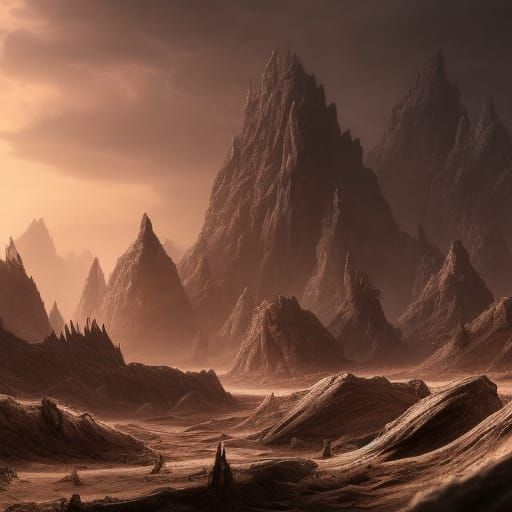This square painting presents an apocalyptic landscape dominated by varying shades of brown and cream, with a slight pinkish hue akin to sepia, but with a more intense vibrancy. The composition is filled with a series of dramatic, steep peaks and pointy, smaller hills that descend in size from the top right corner to the bottom of the image. The tallest and most prominent peaks are located in the top right, gradually giving way to medium and smaller hills in the foreground. The ground, devoid of any vegetation or signs of life, appears barren and almost desolate, with a texture that evokes a sweeping, wave-like effect, merging with the rocky features and enhancing the dramatic atmosphere. The sky is split between a brighter yellowish hue on the left and dark, menacing storm clouds on the right, further casting an ominous overcast across the landscape. This fantastical, surreal vista evokes a sense of desolation and impending doom, with its sharp, jagged formations and eerie, barren ground that appears almost fluid in motion.